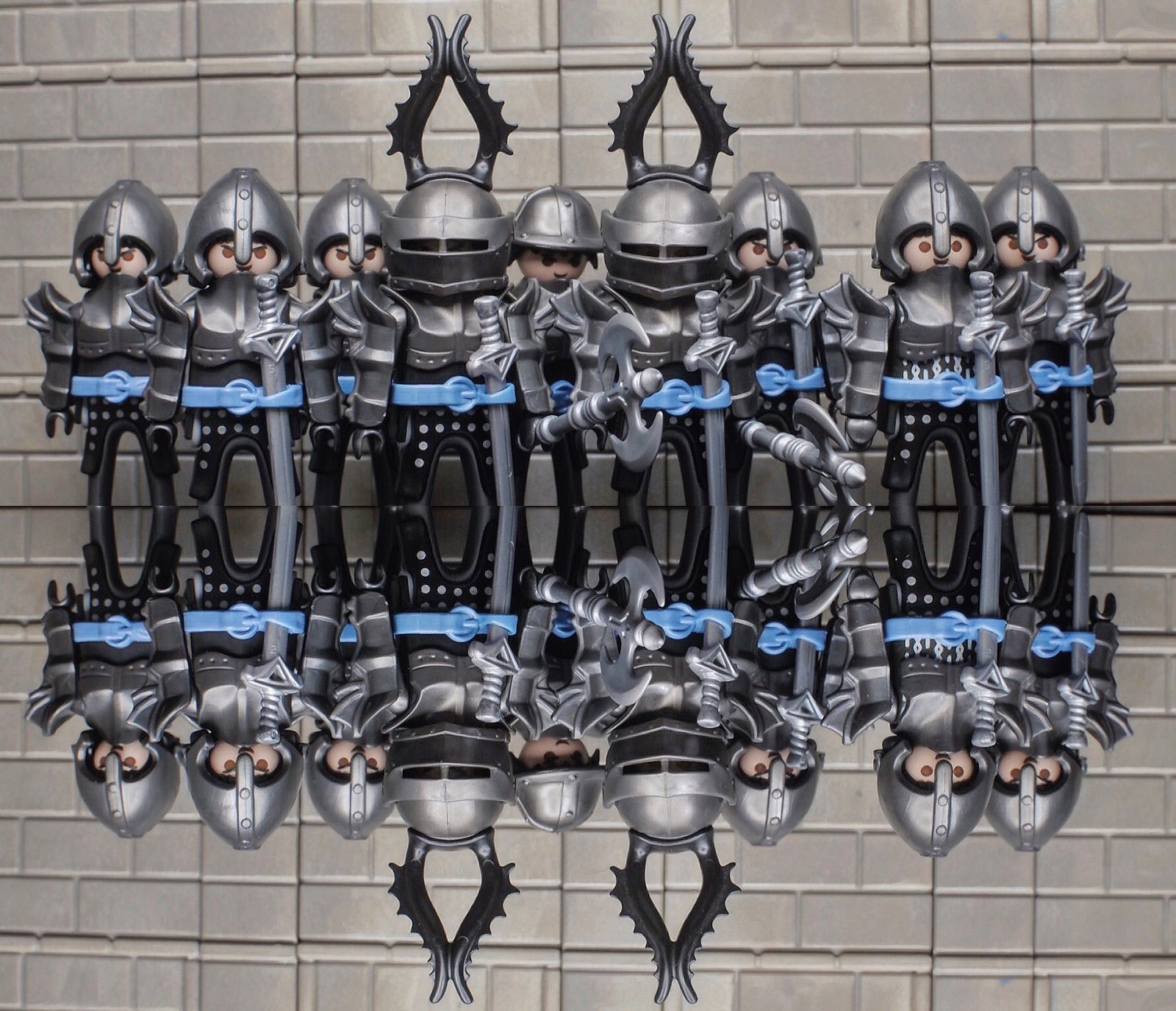The image depicts a collection of toy figurines resembling medieval knights, standing against what appears to be a digitally manipulated backdrop of a gray-colored brick wall, possibly LEGO bricks. These knights, which may be Playmobil or LEGO figures, are captured in a highly detailed and reflective scene. There are a total of nine knights, with seven in the rear and two in the front.

Each knight is clad in detailed medieval armor featuring black chain-link coverings on their legs, gray pants, blue belts, and silver chest plates. All of them wield silver swords, while the front two knights additionally hold double-sided axes. The knights' helmets vary, with some being open-faced, exposing their stern or evil expressions marked by slanted eyebrows and brown eyes, while others wear visored helmets with unique headpieces.

The backdrop of the scene is a textured gray brick wall, subtly accented with shades of tan, pink, and blue, resembling a castle wall. The reflective surface beneath the knights captures their mirror images, adding a sense of depth and symmetry to the composition. This setup gives an impression of a digitally manipulated image, possibly through cropping and reflection techniques, enhancing the medieval theme and the intricate details of the knights.